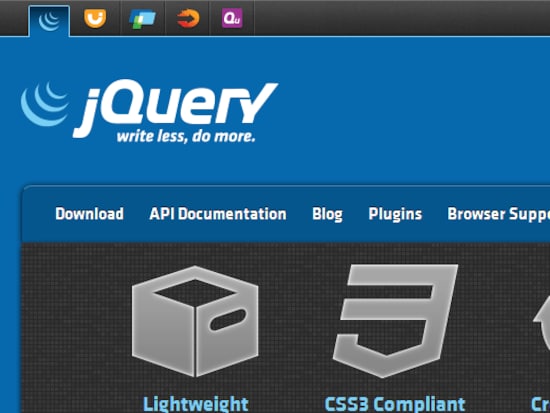This image is a detailed screenshot of a website, likely taken from a laptop in landscape mode. The upper section of the screenshot showcases a typical browser interface with a black tab bar containing five distinct tabs, each with its unique icon. The first tab, which is active and highlighted in light blue, features a logo consisting of three concentric crescent moon shapes in light blue. The second tab displays an icon of an upside-down 'U' within an orange half-oval shape. The third tab has an icon representing layered papers in blue, light blue, and light green colors. The fourth tab features an arrow emerging from a burst, resembling the sun, and the fifth tab displays the letters "QU" inside a purple box.

Below the tab bar, the main content of the page starts with a prominent blue header displaying the word "JQUERY" in large letters, adjacent to the crescent moon icon seen earlier. Alongside this, the slogan "Write Less, Do More" is written against a visually appealing lighter blue background.

Directly beneath the header, a darker blue navigation bar offers several links: "Download," "API Documentation," "Blog," "Plugins," "Browser Support," and others. This section sits atop another segment with a black background, which highlights the words "Lightweight" and a CSS 3 compliant icon presented within a box.

Overall, this screenshot illustrates an overview of the jQuery website, characterized by its clean, user-friendly interface and recognizable branding elements.